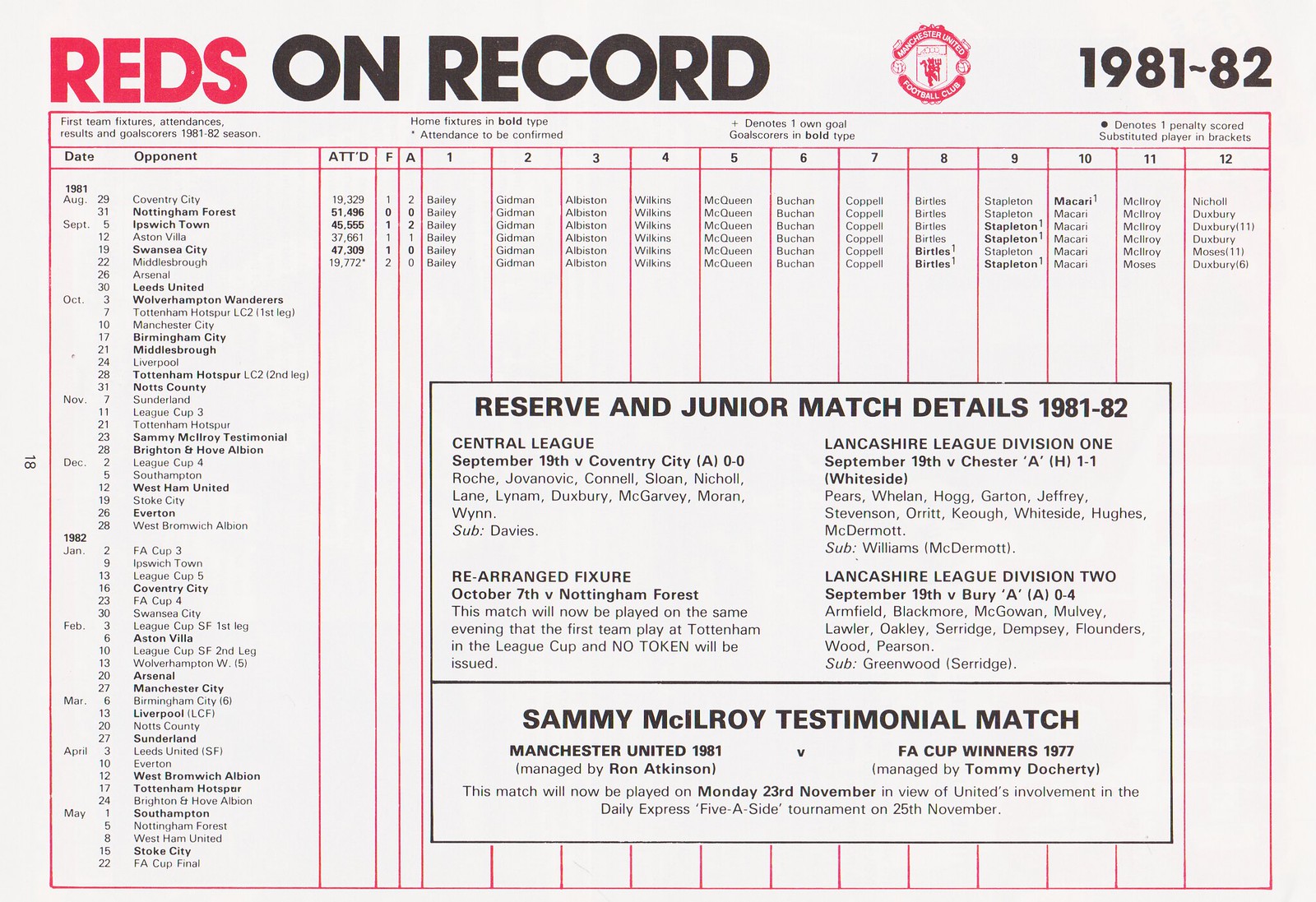This is a detailed photograph of a chart that serves as a roster for a sports team, specifically the Manchester United Football Club, for the 1981-82 season. The background of the image is white with a red-outlined chart prominently displayed in the center. At the top-left, in bold red font, it reads "Reds on Record" with "1981-82" positioned in the upper right corner and a Manchester United Football Club logo at the top-middle.

The chart features various columns and rows filled with black text, detailing essential team information. The top of the chart shows columns labeled as follows: Date, Opponent, ATTD, F, A, and then numbers 1 through 12. This table is filled with data up through the month of September.

On the column headers, there is a legend clarifying what each symbol means, such as home fixtures in bold, attendance to be confirmed, denotes one own goal, goal scores in bold, denotes one penalty scored, and substituted player in brackets.

Midway down the chart, there's a bold black-outlined box titled "Reserve and Junior Match Details 1981-82" that provides additional match details. Below this, another smaller box reads "Sammy McIlroy Testimonial Match," offering specific details regarding this commemorative game.